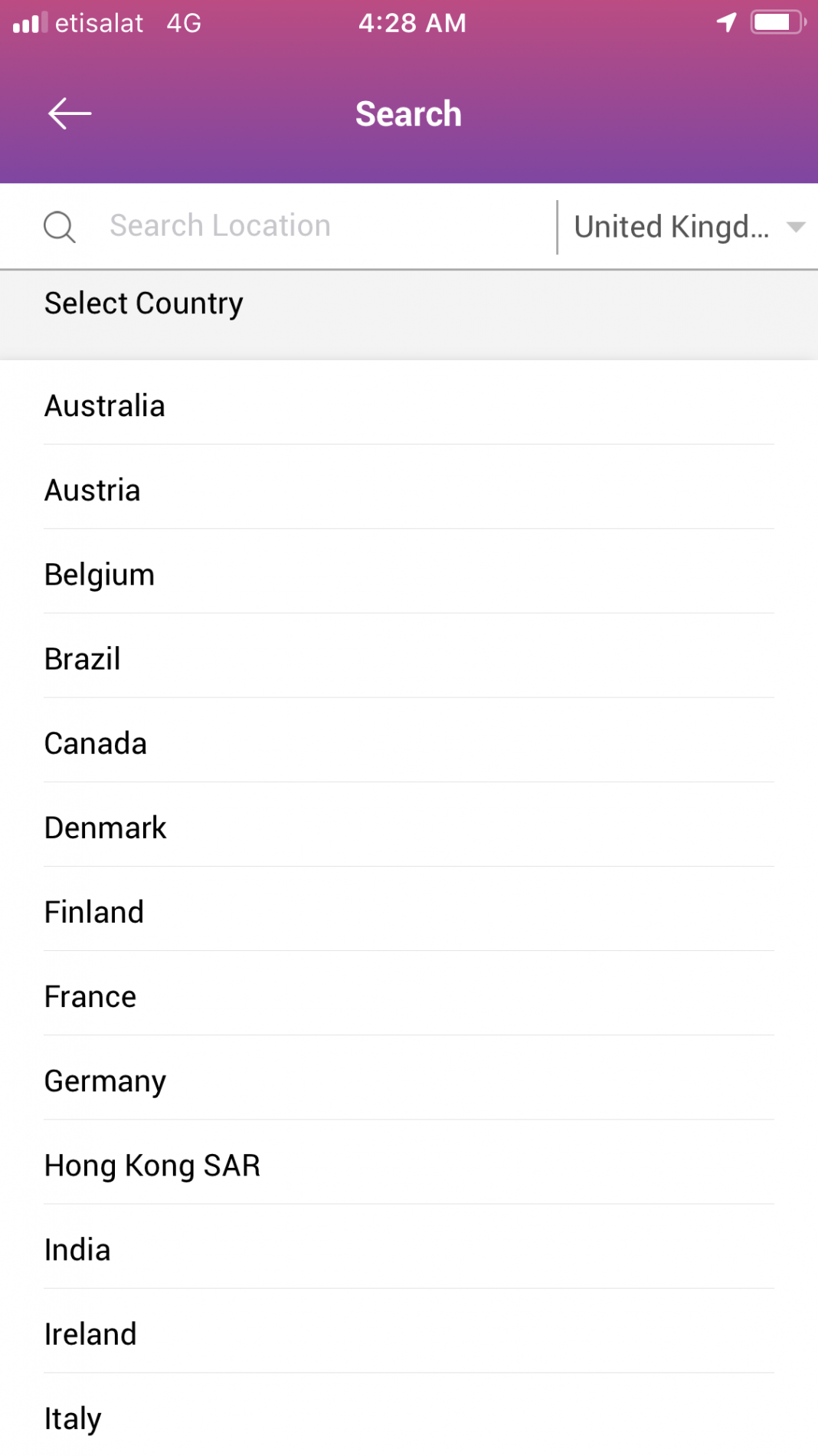The image appears to be a screenshot from an electronic device, depicted at 4:28 AM with a purple background. The status bar at the top indicates a nearly full battery, with 75% charged, and the device is connected to a 4G network. 

Prominently displayed is a search bar, rendered in white, accompanied by a left-pointing arrow. Adjacent to the search bar is the label "Search location / United Kingdom" and an option to select a different country.

Below the search input, a vertical list of countries is visible on the left side, starting with Australia and progressively including Austria, Belgium, Brazil, Canada, Denmark, Finland, France, Germany, Hong Kong S.A.R., India, Ireland, and concluding with Italy.